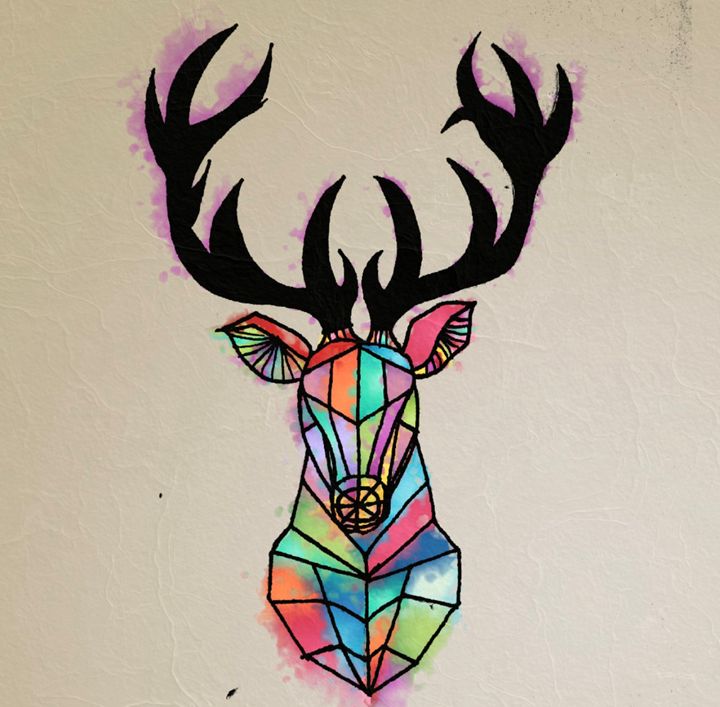This is a detailed watercolor painting of an elk's head and neck, stylized with vibrant geometrics and dynamic colors. The artwork, created on cream-colored paper, presents the elk almost symmetrically from a frontal perspective. The black antlers stand out with hints of purple stains around them, creating a striking contrast against the vividly colorful face and neck, which are composed of various shapes. The watercolor technique gives it a melting effect, as if the colors—ranging from light blue, orange, purple, yellow, pink, and red—are sinking into the paper, almost glowing. The entire piece exudes creativity and meticulous detailing, with a background that blends into the beige wall, enhancing the elk’s bold and artistic representation.